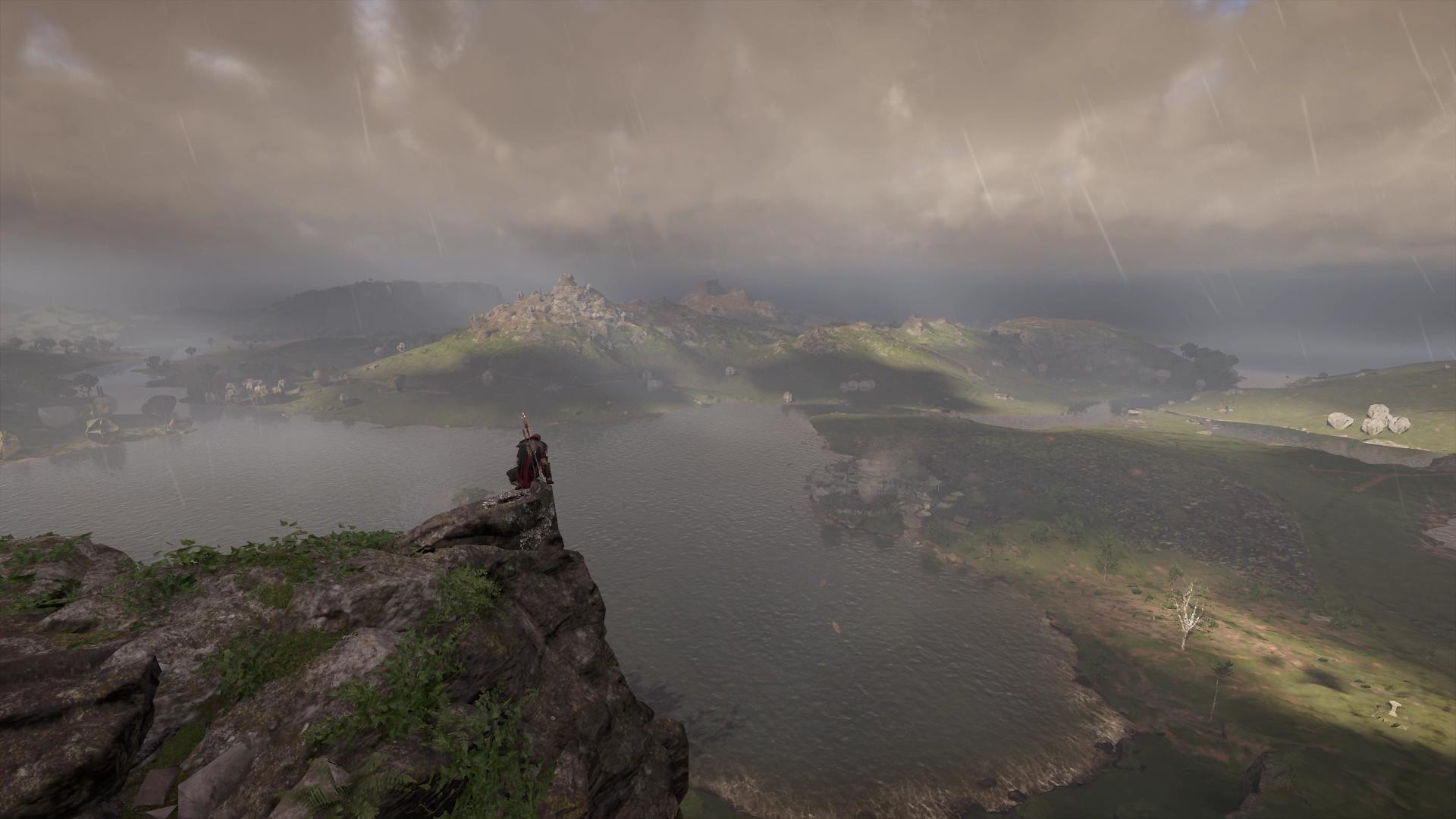The image is a detailed screenshot from a realistic modern-style game, depicting a dramatic scene set in a rugged, medieval landscape. A man, clad in a black cloak with two swords strapped to his back, stands or crouches precariously on a steep, sturdy cliff's edge. He seems to hold a staff or another weapon in his left hand. The rock, dotted with small patches of green vegetation and weeds, juts out above a vast, rough lake nestled in a valley below. 

In the background, there are several hills and mountains covered in trees and small bushes. A small town with white buildings can be seen near the lake, to the right of where the man stands. The weather is dark and rainy, evidenced by the cloudy sky and visible raindrops falling. 

A dramatic play of light illuminates the scene: an opening in the clouds at the top left corner casts a beam of light down to the bottom right, highlighting a small area of the valley floor. In the distance, hints of more rugged terrain and possibly stone structures or castles add to the old-fashioned medieval atmosphere. The perspective suggests that the camera is suspended in the air, perhaps 10 meters away, capturing this cinematic and perilous moment from behind the character.